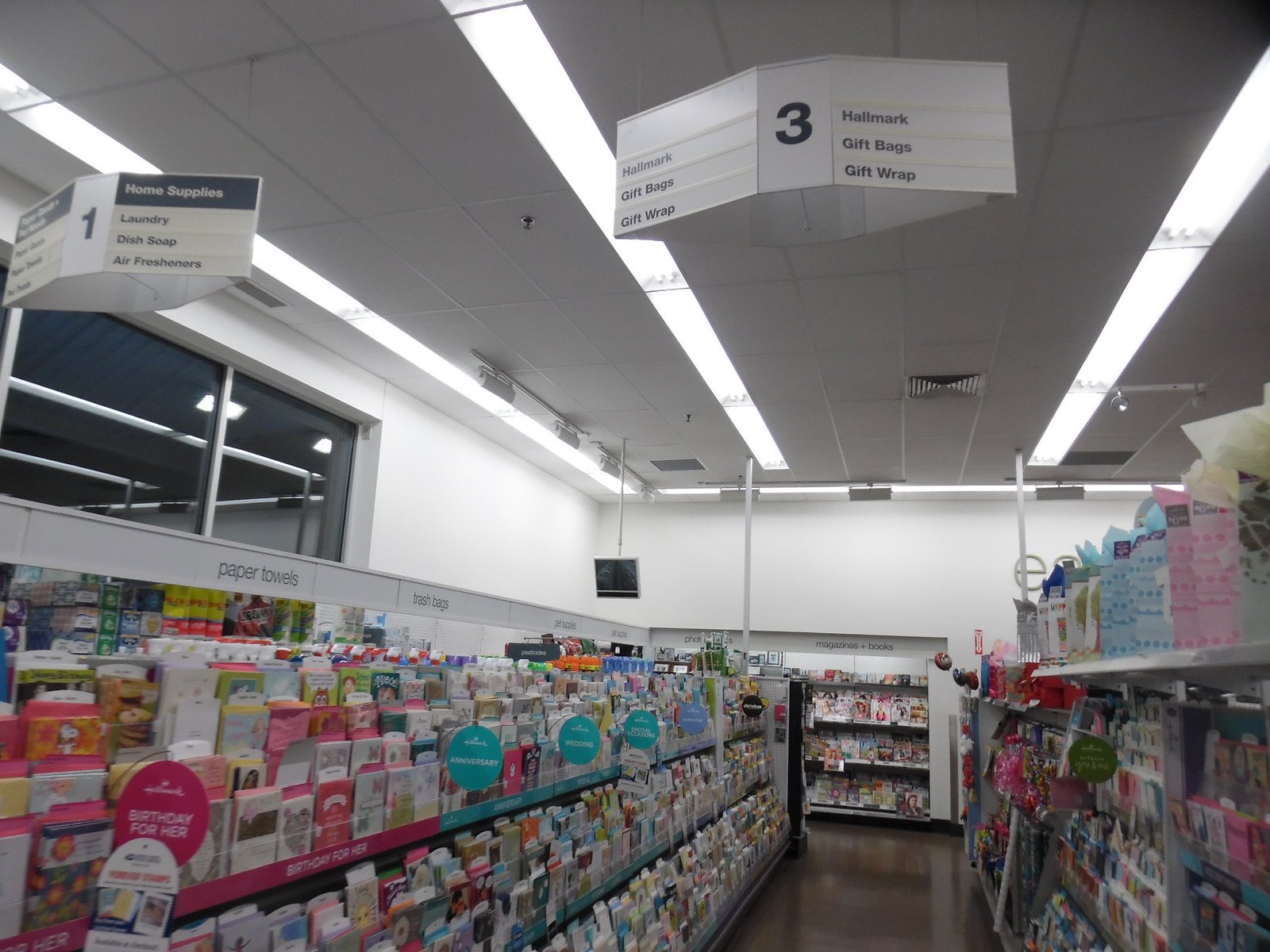This image depicts a greeting card aisle, likely inside a drugstore, characterized by a drop ceiling with white tiles and fluorescent lights. The aisle, labeled as Aisle 3 with a white hanging sign, displays sections for Hallmark, gift bags, and gift wrap. The left side of the aisle features a lengthy rack lined with various greeting cards spanning multiple rows, vividly colored in whites, pinks, and blues, designated for different occasions. On the right side, there are additional cards and a shelf exhibiting gift bags and tissue paper, with wrapping paper and bows towards the back. The floor appears brown, possibly due to reflections from the lighting. In the background, a magazine rack is visible, along with a sign for Aisle 1 denoting items like home supplies, laundry, dish soap, and air fresheners. Additionally, a security monitor hangs in the back left corner, and a band along the shelves lists paper towels. Two high windows are positioned on the left wall, providing a sense of depth and structure to the scene.